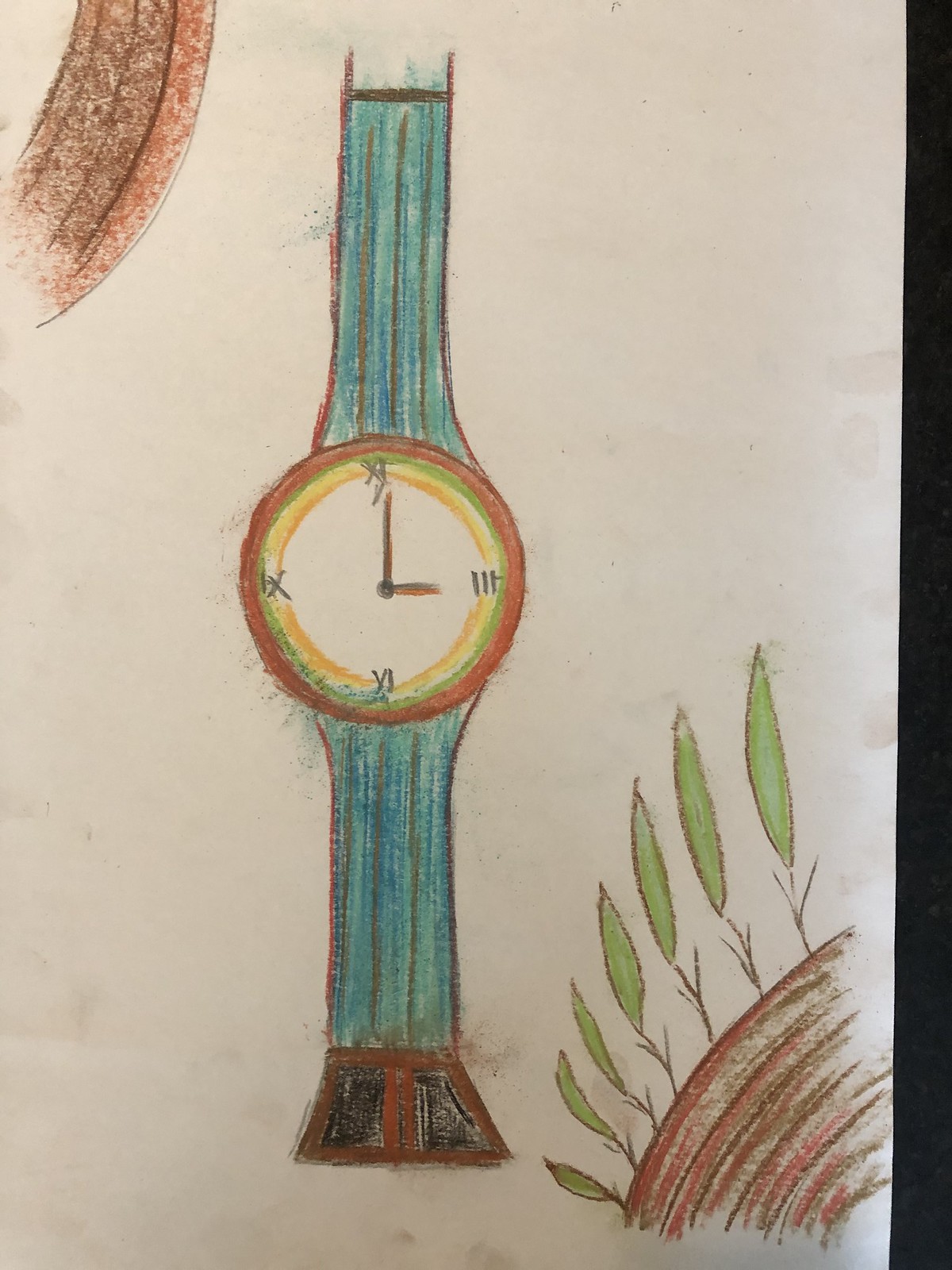The image depicts a meticulously hand-drawn wristwatch, likely crafted with colored pencils and possibly some crayon. The off-white background sets off the detailed artwork. The wristwatch itself features a teal wristband with brown stripes and a brown latch. The circular watch face is framed by a brown border and displays Roman numerals at the 12, 3, 6, and 9 positions in black. The watch hands are brown, with a black screw connecting them at the center, indicating the time as three o'clock.

The face of the watch is artistically colored with concentric circles of yellow and green. Surrounding the watch face is a mixture of light and dark brown, with some burgundy tones suggesting a curved, landscape-like design, resembling a farmer's field. To the right, a semicircle of varying shades of brown houses brown stems that lead to green leaves, giving a naturalistic touch. The bottom-right section of the drawing features a design reminiscent of rushing water, accompanied by single-leaf plants emerging from it, enhancing the image's overall organic feel. The entire piece displays a great deal of care and creativity, making it a captivating and detailed work of art.